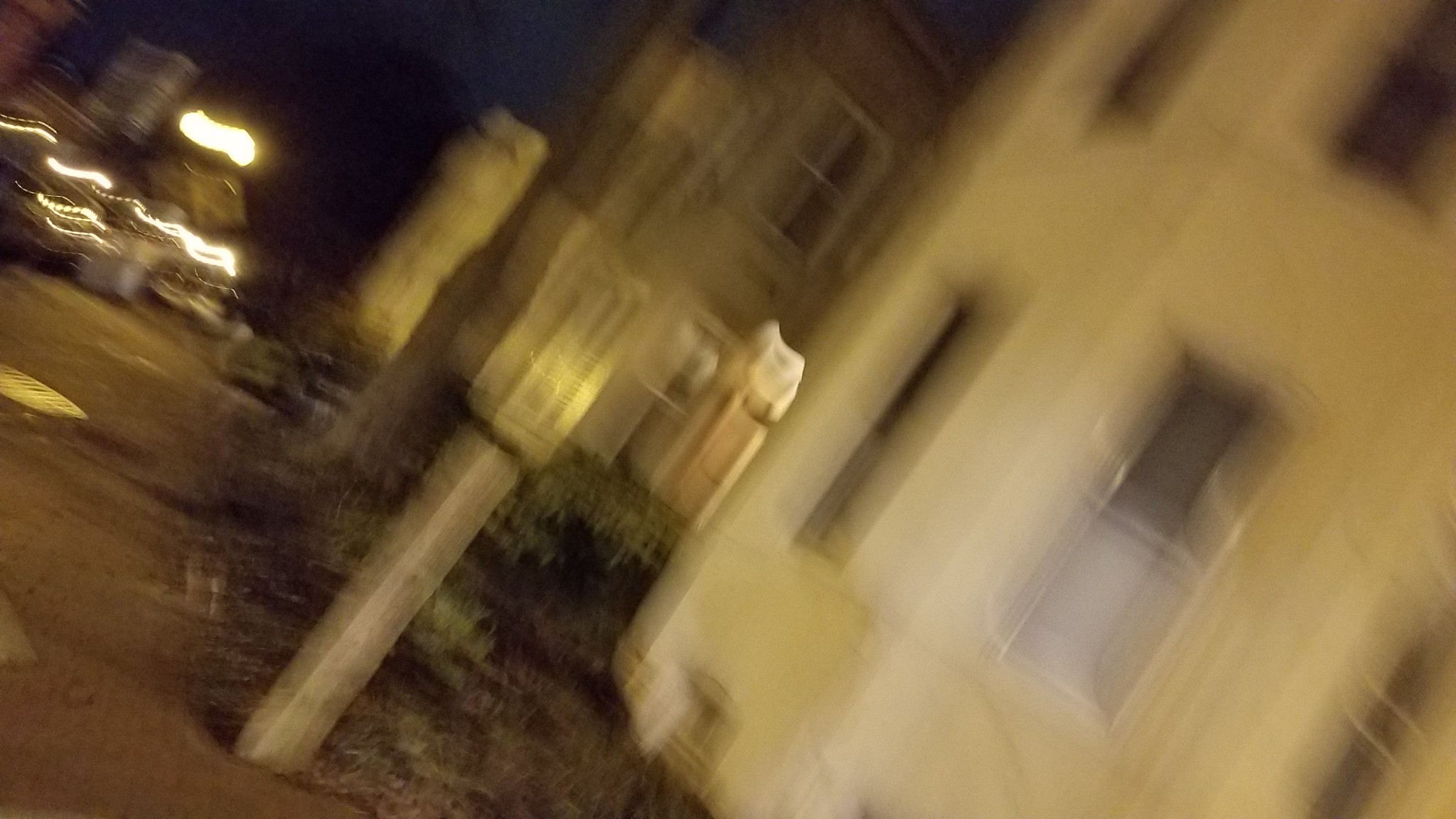This is a blurry nighttime photograph taken at a canted angle, depicting an outdoor scene with both residential and commercial elements. In the foreground, there are two apartment buildings. The one to the right appears to be white or creamy stucco with four visible double-hung windows, and the other, slightly obscured by the angle, is made of brick with some white windows. Both buildings are adorned with lampposts and shrubbery, and a gray post is seen in front of the white building. The slanted perspective makes the structures seem tilted from left to right. Further down the sidewalk, numerous squiggly lights suggest the presence of shops or restaurants, indicating a lively, illuminated area in the distance. The overall composition hints that the photo was captured on a sidewalk within a mixed residential-commercial neighborhood.